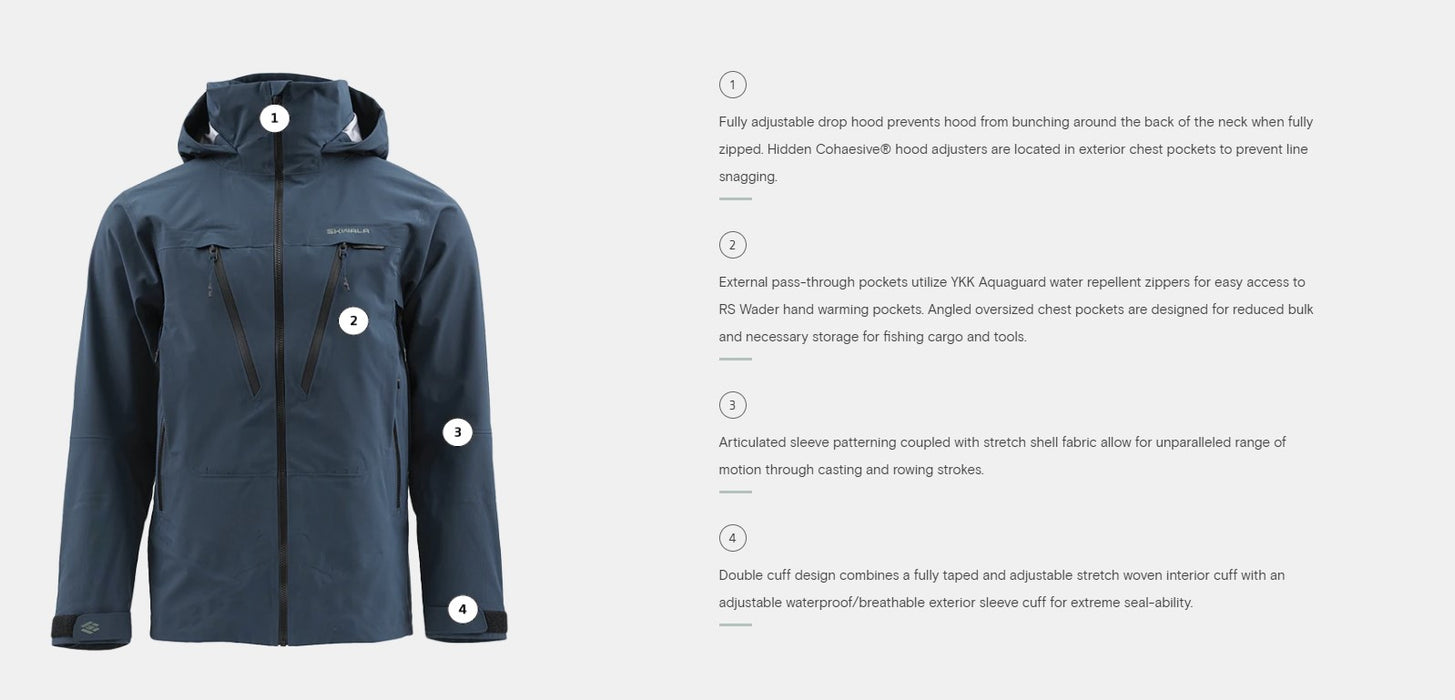This image is a detailed advertisement for a dark navy blue waterproof jacket available on an online store, showcasing various features of the garment. The jacket, made from a water-repellent material, includes a fully adjustable drop hood designed to prevent bunching around the neck. Hidden cohesive hood adjusters are located in the exterior chest pockets to avoid line snagging. The central zipper is flanked by two diagonally-angled chest zippers featuring YKK AquaGuard water-repellent technology, ideal for easy access to hand-warming pockets and essential fishing tools. The jacket also boasts articulated sleeve patterning coupled with a stretch shell fabric, providing an unparalleled range of motion for activities like casting and rowing. Furthermore, the design includes a double cuff system combining an adjustable, stretch-woven interior cuff and a waterproof, breathable exterior sleeve cuff, ensuring extreme sealability against water. The image labels these features with white numbered circles that align with descriptive text, enhancing the comprehensibility of the jacket's advanced functionality.